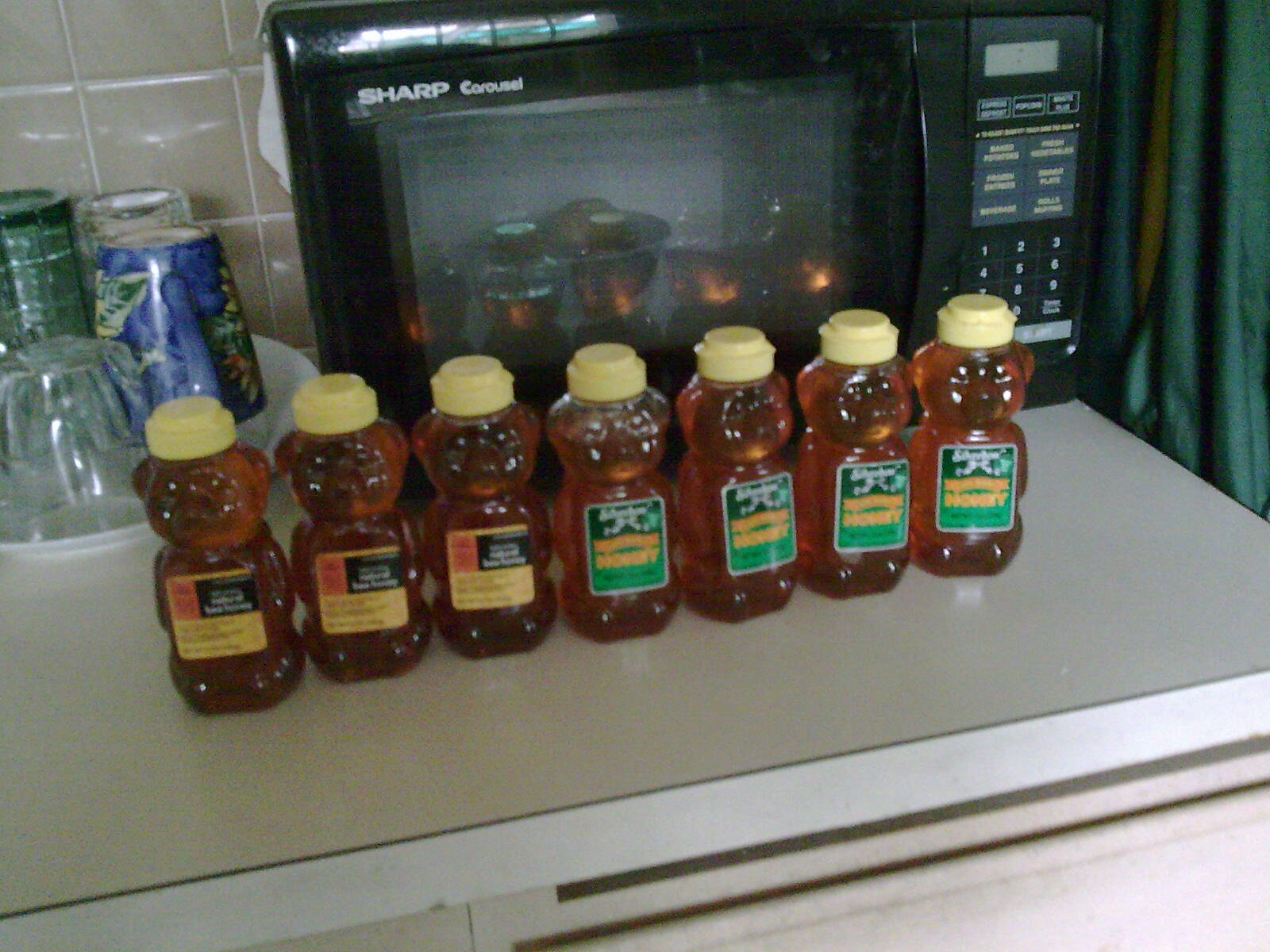The image depicts seven clear plastic bear-shaped honey jars, each filled with golden-brown honey and sealed with yellow caps. The honey jars are neatly arranged on a pristine white kitchen countertop. The three jars on the left feature yellow labels with black and red details, while the four jars on the right have labels in varying shades of green and white text. Positioned behind these jars is a black Sharp Carousel microwave, with its see-through glass door revealing a white pattern on the right side of the image. To the left side of the image, there is a plate holding an assortment of glassware, including a transparent glass, a green glass, and a blue ceramic mug adorned with yellow and green floral designs, all placed upside down. The scene is set against a subtle background of kitchen tiles and dark green curtains, enhancing the domestic ambiance.